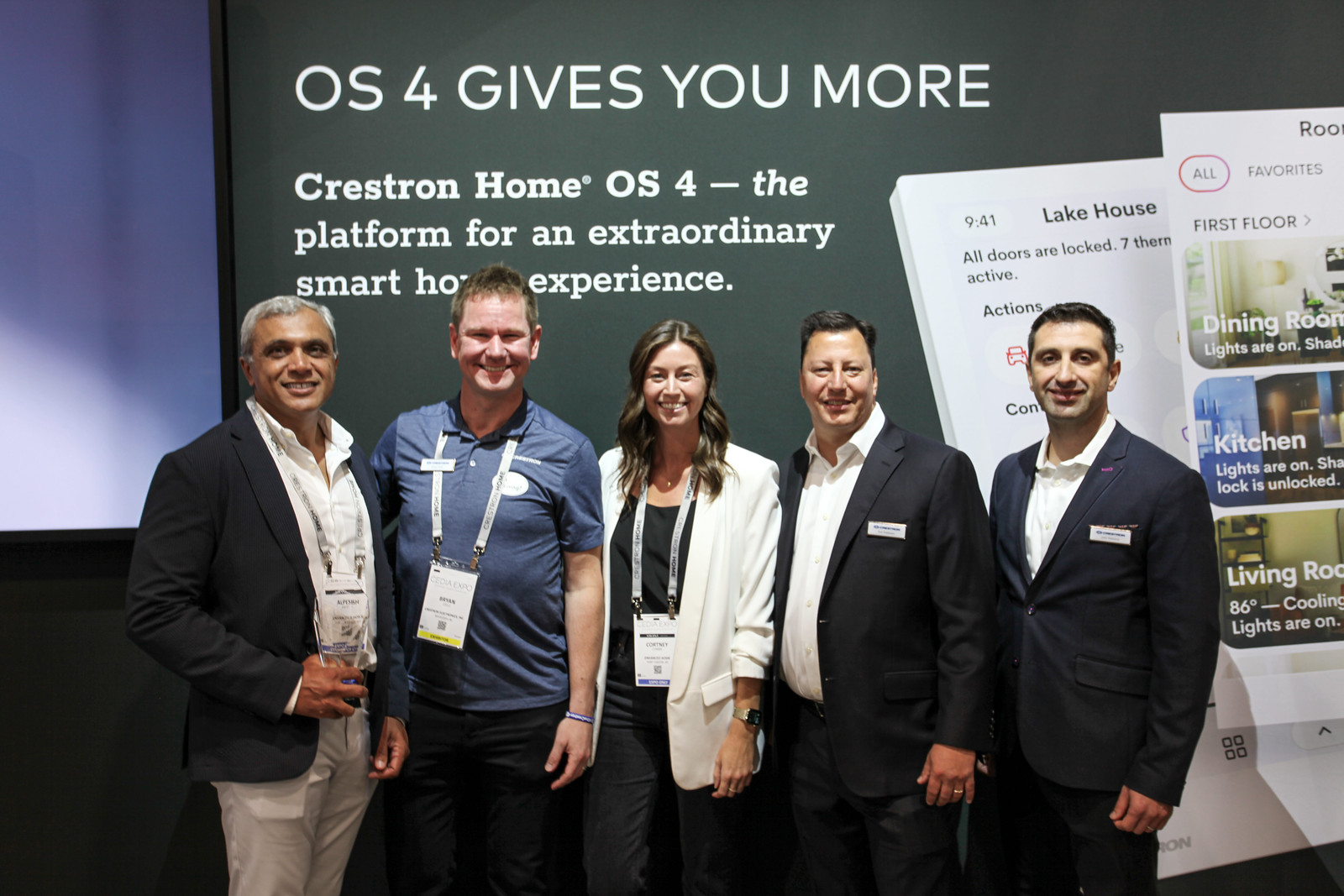This photograph features a group of five professionals at a conference, with a businesswoman in the center flanked by four men. The woman is dressed in a white jacket over a black shirt and black pants. To her immediate left is a man in a blue t-shirt and black pants, both sporting lanyard ID badges. To his left stands a man with darker skin and gray hair, dressed in a white shirt, black suit jacket, and tan pants, also with an ID badge around his neck. To the woman's right are two men, both wearing black jackets, white undershirts, and black pants, with their name tags inserted in their jacket pockets. The group is posing in front of a predominantly green sign that reads "OS4 gives you more" at the top, with "Crestron Home OS4, the platform for an extraordinary smart home experience" beneath. The setup suggests they are part of the event or company related to the conference.